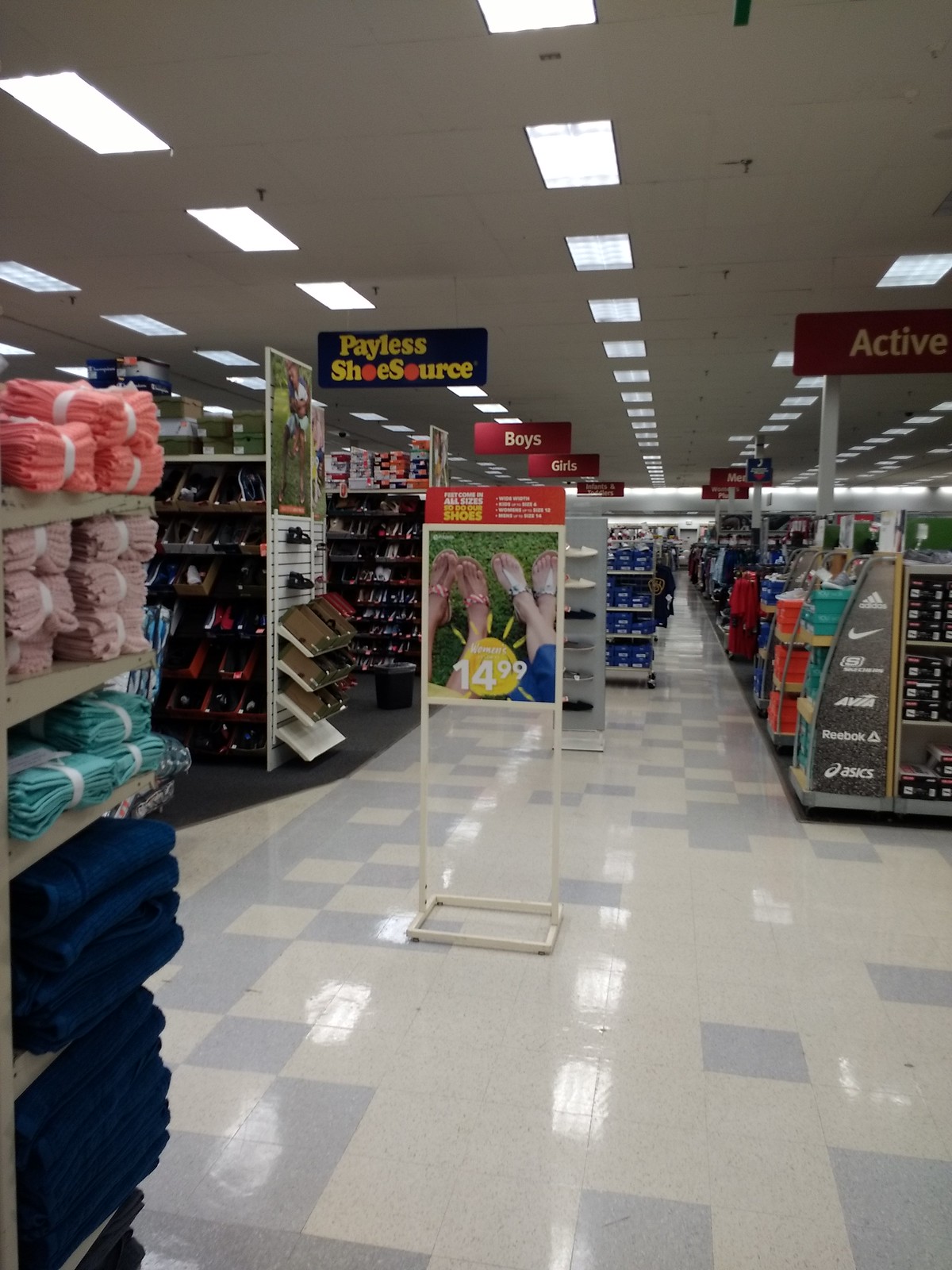This photograph captures the interior of a large Payless Shoe store, featuring a white ceiling with uniform rows of flat, fluorescent lights. The floor is a mix of white and blue tiles, seemingly arranged in a random pattern. Central in the image is a hanging sign from the ceiling that reads "Payless Shoe Source" in yellow letters against a blue background. Another sign on the right side spells out "Active" in white font on a red background. The store is well-stocked with numerous aisles filled with shoes, some in boxes and others displayed openly. To the left, shelves hold various textiles, possibly washcloths, towels, and possibly socks in pink, peach, green, and blue hues. In the foreground, a sign on a holder prominently displays a price of $14.99.